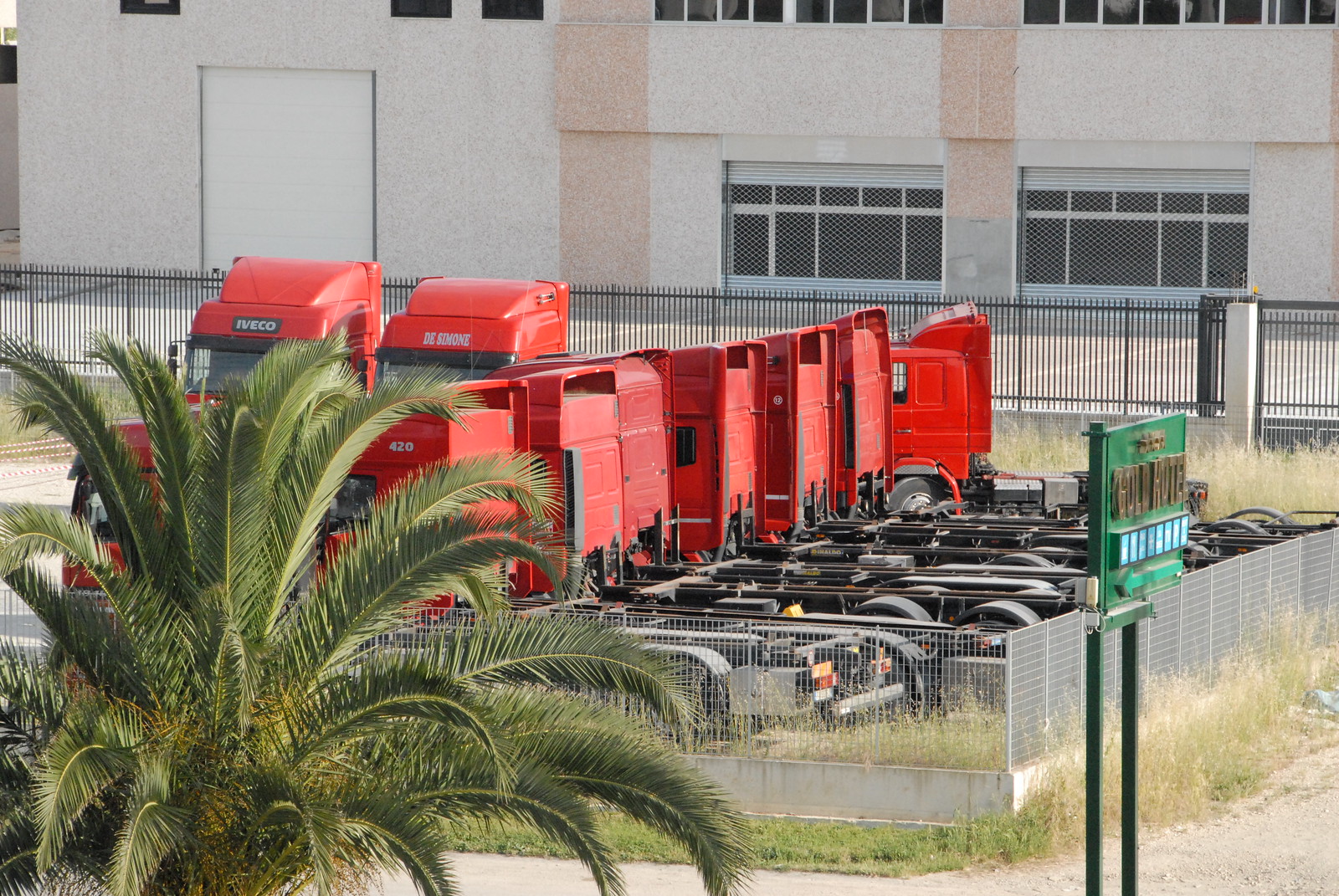The image depicts a small parking lot containing around 8 to 10 red Iveco big rigs, all appearing identical and without any trailers attached. These trucks are fenced in by a chain-link fence, with a black steel fence and a large grey and cream building featuring various windows visible behind them. In the foreground to the right, there's an unreadable green sign on black poles, which some believe possibly reads "Gold Hotel" with additional text likely indicating vacancy status. The lower left corner of the image shows a palm tree, obscuring part of the view of the trucks. The area around the parking lot is surrounded by neglected grass and patches of brown dirt, suggesting a lack of maintenance.